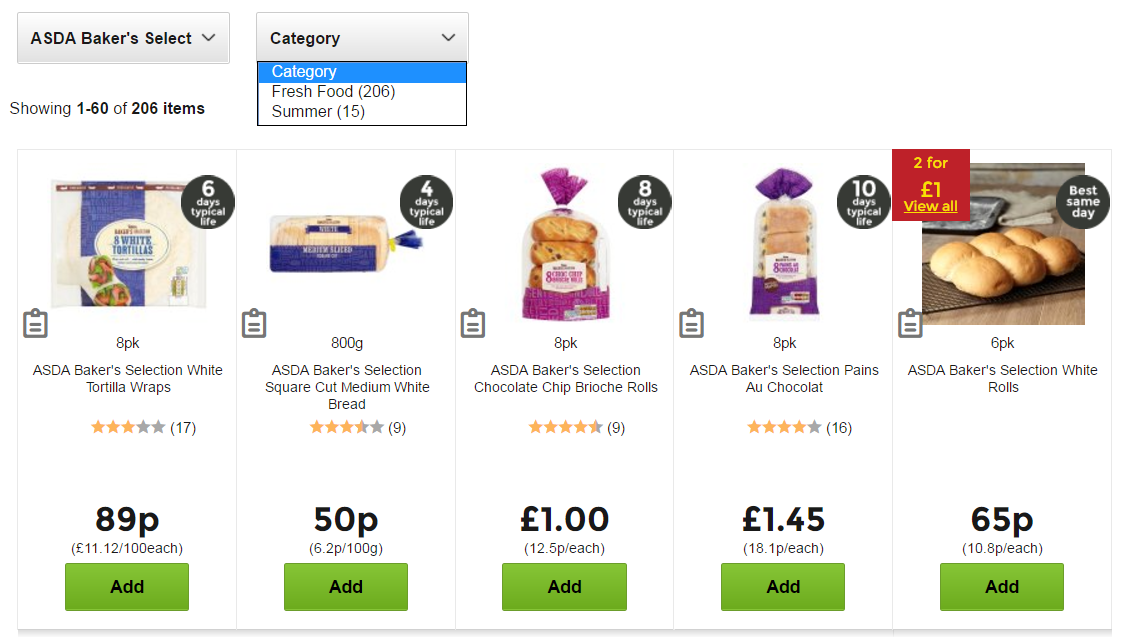A partial view of an online grocery shopping website, showcasing a selection of food products available for purchase. The interface displays a couple of drop-down menus titled "ASDA", "Baker's Select", and "Category," although no specific filters have been applied yet. Visible products include:

1. **Baker's Selection White Tortilla Wraps** - Priced at 89 pence, featuring a typical shelf life of six days.
2. **Square Cut Medium White Bread**.
3. **Chocolate Chip Brioche Rolls** - Priced at 1 British pound.
4. **An unspecified chocolate item**.
5. **Additional white rolls**.

Each product is shown with a corresponding picture and price, all listed in British pounds or pence. "Add" buttons are available beneath each price for convenient selection. Some product images also display additional information such as shelf life or expiration dates.